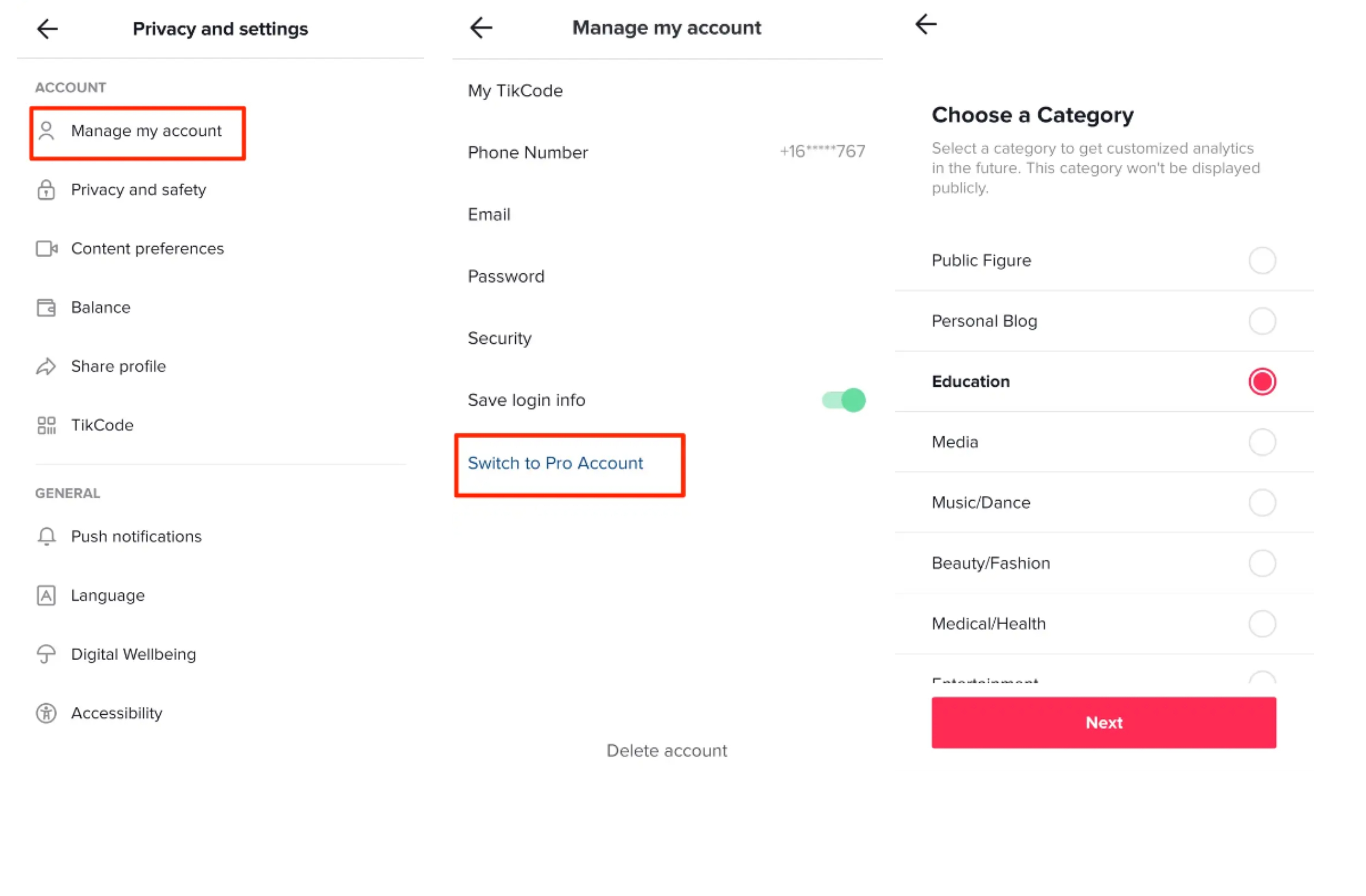In the top left corner of the image, there is a gray arrow pointing to the left, accompanied by the text "Privacy and Settings." Directly below, the word "Account" is prominently outlined in a red box, with the subheading "Manage My Account" beneath it. Moving down the list of choices, the categories include: Privacy and Safety, Content Preferences, Balance, Share Profile, TikCode, Push Notifications, Language, Digital Well-being, and Accessibility.

On the right side, the text "Manage My Account" reappears, with options listed below it: My TikCode, Phone Number, Email, Password, Security, and Save Login Info. Positioned to the right of these options, there is a green circle. Further down, another option outlined in a red box is "Switch to Pro Account." To the far right, there is a section titled "Choose a Category." The available categories listed underneath are Public Figure, Personal Blog, Education (highlighted in black), and to the right of "Education," a red circle is visible. Further categories include Media, Music, Dance, Beauty, Fashion, Medical, and Health.

At the bottom of the rightmost column, there is a long red rectangle containing the word "Next" in white text.